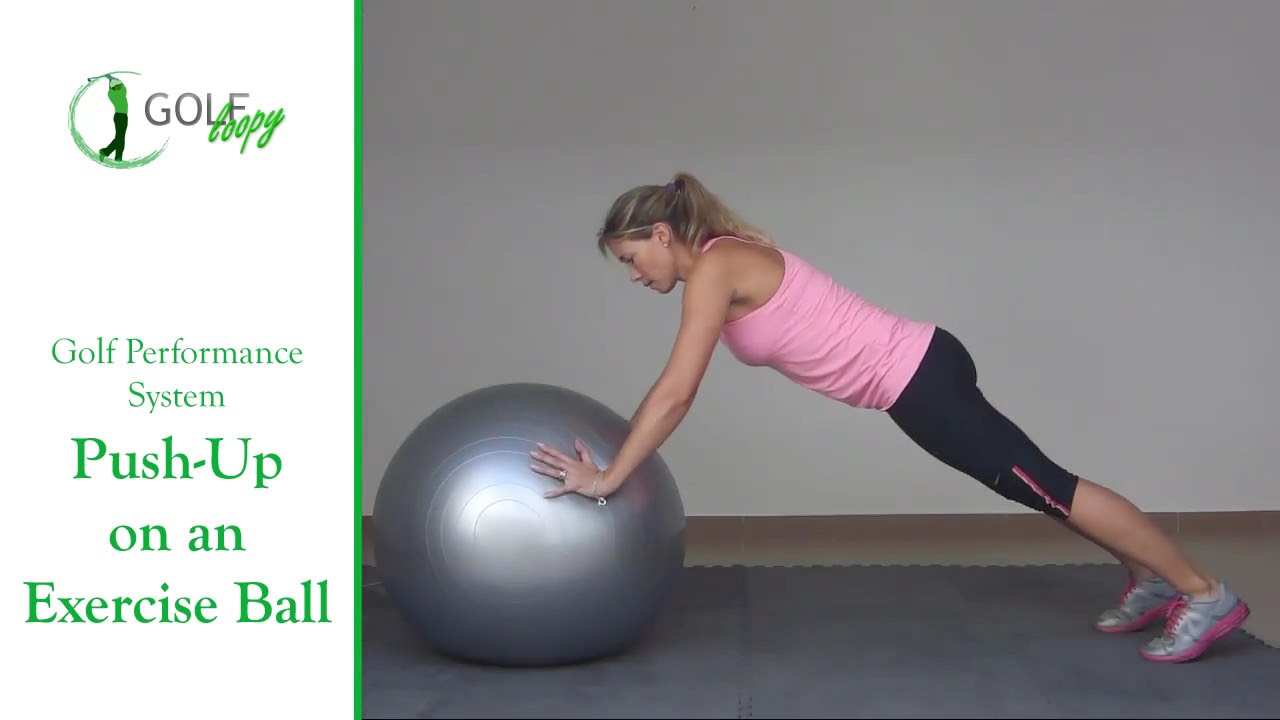The image features a fitness scenario split into two distinct sections. On the left third of the image, there is a white background with text and graphics. At the top, the text reads "Golf Happy" with "Golf" in black and "Happy" in green cursive letters. Below this, there is an illustration of a man swinging a golf club, depicted with a green arc indicating the swing's path. The golfer is dressed in a green shirt, black pants, green shoes, and a white hat. Below the golfer, the text says "Golf Performance System Push-up on an Exercise Ball," all in green letters.

To the right of this text section, the image showcases a woman engaged in a fitness routine, specifically performing a push-up on a gray, reflective exercise ball. She leans diagonally towards the left, maintaining a plank position. The woman has dark hair with blonde highlights tied back and wears a pink, sleeveless workout tank top, black knee-length exercise pants featuring a pink stripe, and silver and pink shoes. Her hands press into the ball, causing a visible indentation due to the applied pressure. She is positioned on a black mat atop a brown, tiled floor, set against a light gray wall. The overall environment suggests an indoor fitness class or personal workout session.